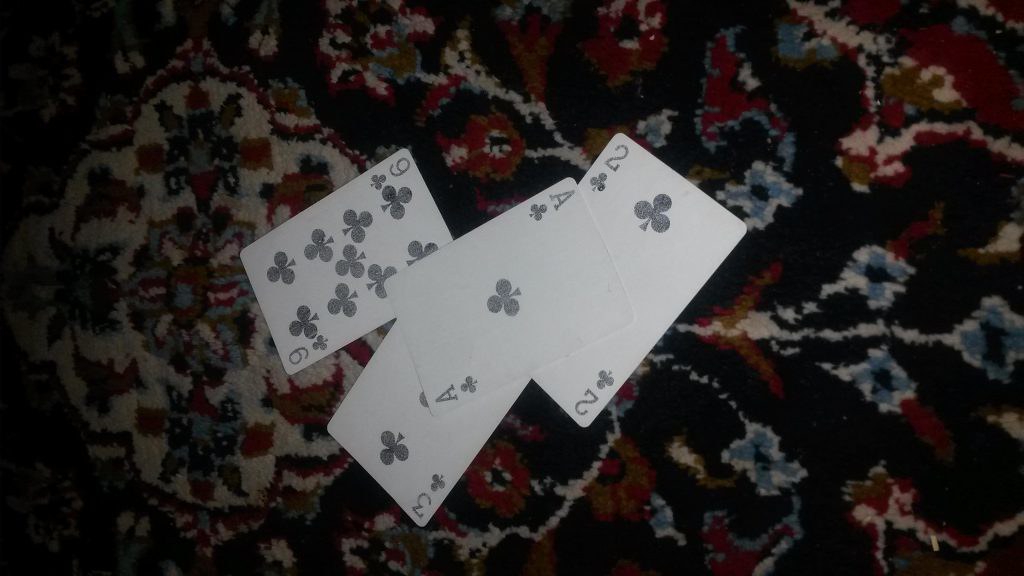The image depicts four playing cards placed on a patterned carpet. On the left side, there's the Nine of Clubs, followed by the Ace of Clubs directly above the Three of Clubs. Adjacent to these, on the right, is the Two of Clubs. All cards are oriented towards the top-right corner of the image. The carpet features an intricate design: on the right side, it shows blue and red flowers, while on the left, there's a larger, four-petal flower with a mostly white background and blue flowers surrounded by red petals. The center of this larger flower is dominated by a blue segment surrounded by a mix of red, white, blue, and green hues. The remaining background of the carpet is black, creating a stark contrast against the vibrant floral patterns. The scene appears to be captured at night.